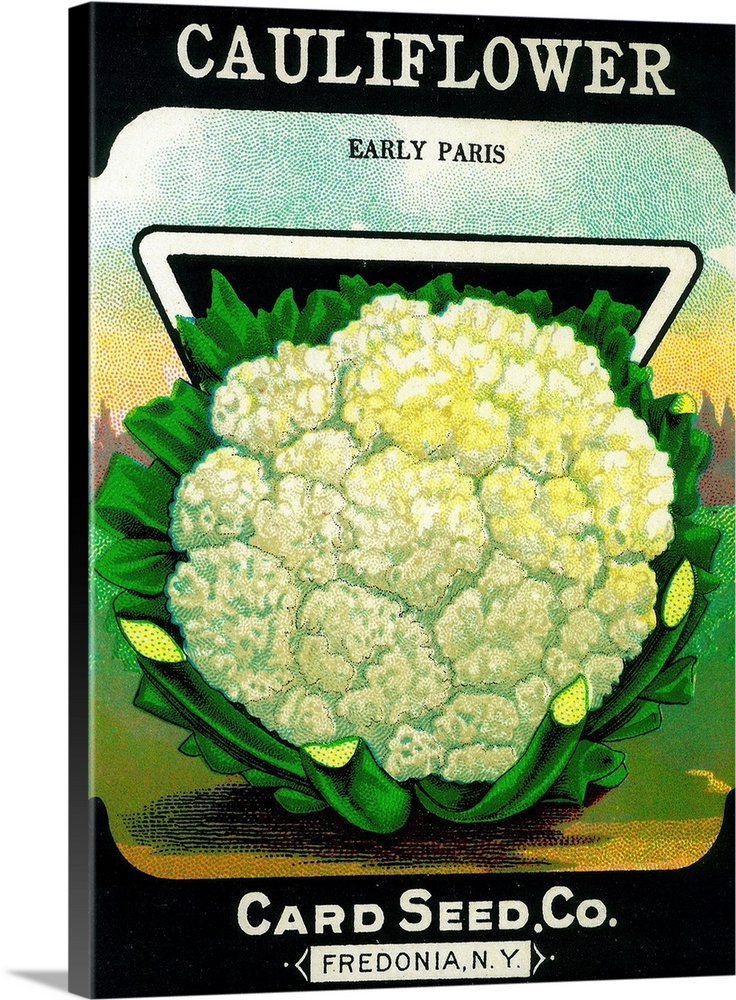The advertisement image showcases an exquisite, full head of cauliflower prominently displayed on a black background. The image is centered within a rounded-edged square featuring a gradient that transitions from white at the top to yellow, then to various shades of brown, green, and black towards the bottom. At the top of the image, "Cauliflower" is boldly written in large white letters. The cauliflower itself glows with a bright white hue, punctuated by subtle hints of yellow, framed perfectly by its verdant green leaves which have been partially cut away to reveal the vegetable in all its glory. The intricate details of the leaves and the inner lighter green stalks are captured vividly, adding texture and depth. At the center of this captivating image, "Early Paris" is inscribed, highlighting the variety of the cauliflower. At the bottom, the advertisement features the text "Card Seed Co., Fredonia, N.Y." in white lettering, situating the source of this appealing produce. The entire composition is set against a contrasting black backdrop, enhancing the vibrant colors of the cauliflower and its surrounding greenery.